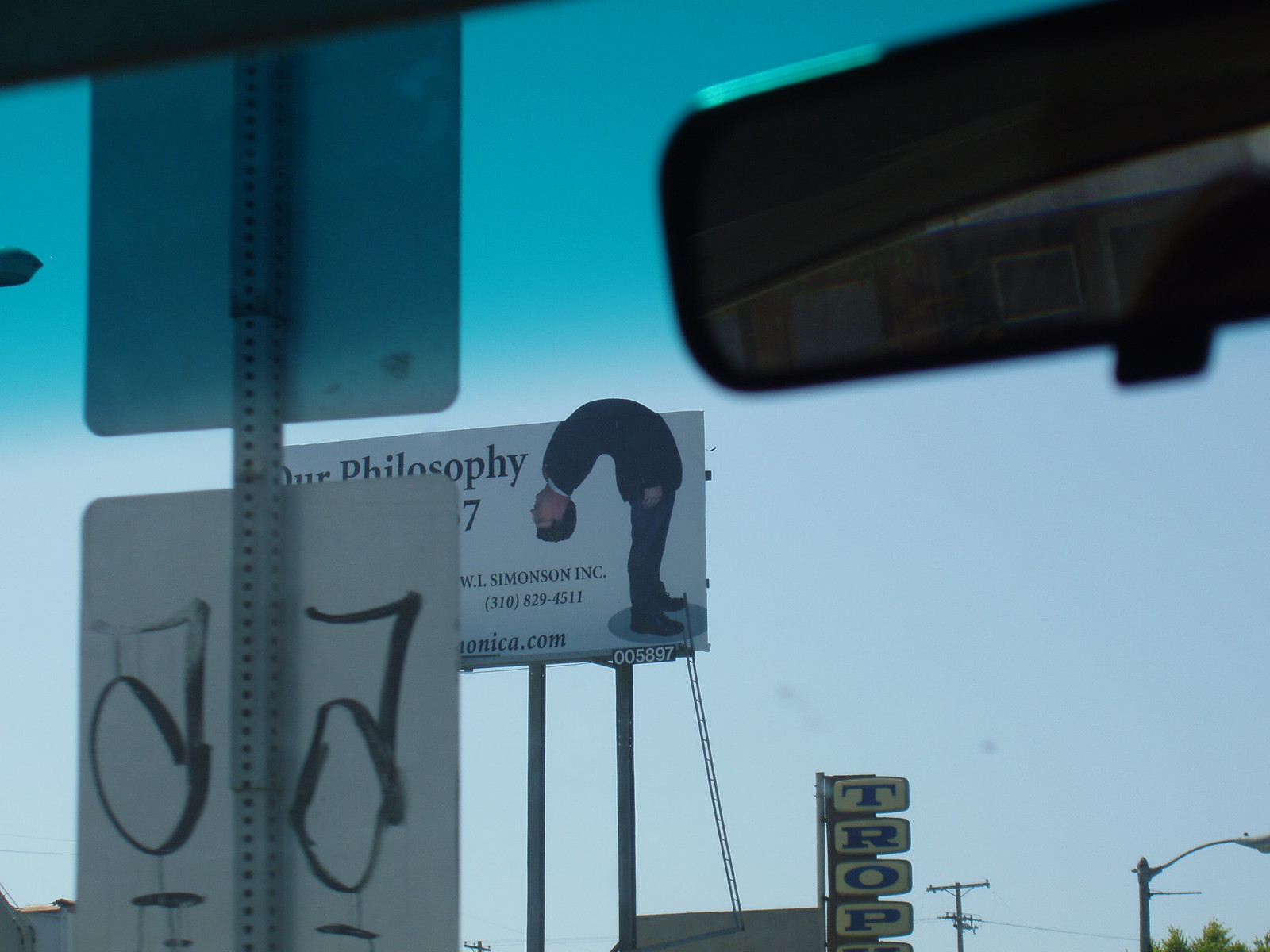The photograph, presumably taken from inside a car, captures a scene through the windshield. The windshield itself has a noticeable dark blue tint along the top edge, and the black rearview mirror is visible on the right. On the left side of the frame, a street sign mounted on a perforated gray pole stands out. This pole supports two vertically aligned rectangular signs viewed from their backsides. Both signs have been defaced with spray paint or marker, displaying a distinctive symbol resembling a '7' with a circle beneath it.

In the background, a partially obscured billboard adds an element of mystery. The billboard, set against a white backdrop, prominently features the text "Our Philosophy" followed by a barely legible number '7.' The name "WI Simonson Incorporated" and a phone number are also partly visible.

Adding to the peculiar scene, a man dressed in a suit is bizarrely bent over at the waist, with his head hanging unnaturally low, even below his rear. He stands rigidly on a small circular rug, as if frozen in an impossible pose. Beneath him, a snippet of another sign reads "TROP," completing the unusual tableau captured through the car's windshield.